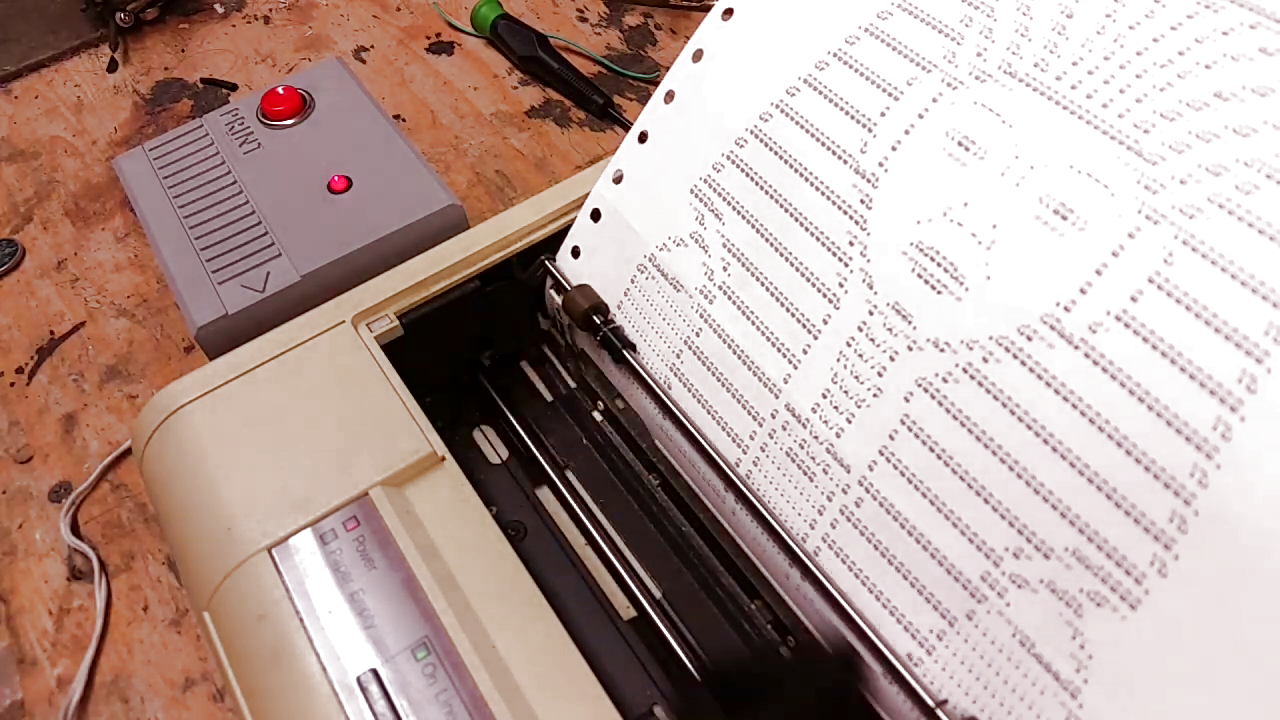The image features an old beige dot matrix printer, prominently placed in the center of the scene, reminiscent of models popular in the 1980s. It has a sheet of paper flowing out, adorned with the characteristic punched holes on the sides, indicating the use of a tractor feed mechanism. The printout itself depicts an Egyptian pharaoh, likely King Tutankhamun, characterized by a headdress and distinct beard, rendered in a crude, symbolic dot matrix style.

Adjacent to the printer, there is a gray device with a conspicuous red button and a glowing light labeled "Print." Below this button, vertical gray lines are apparent. The printer and its enigmatic companion device rest on a heavily stained wooden work table, which is scattered with bits of dirt and some unknown tool or cable with a green tip. This setup suggests a vintage computer workstation, echoing the bygone era of early personal computing technology.